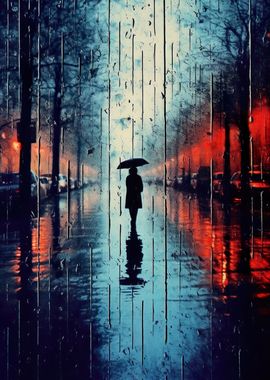The poster depicts a rainy evening street scene with a solid black silhouette of a woman standing alone in the middle of the street, holding an umbrella. The woman, who appears to be wearing a dress or a mid-thigh coat, casts a mirrored reflection on the wet pavement. The sky is dark with a bluish glow at its center, enhancing the melancholic mood. On either side of the street, trees and parked cars are visible, while buildings nearby are illuminated in reddish-orange hues, casting their reflections onto the wet pavement. The street flows with textures of lines, emphasizing the heavy rainfall and the deserted, lonely atmosphere.